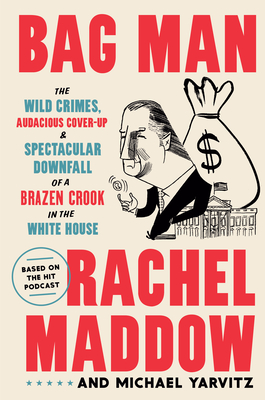The image appears to be an advertisement or book cover for "Bag Man" displayed on a beige background. At the top, large, bold red letters spell out "Bag Man," with an additional tagline below, in various colors, stating, "The Wild Crimes, Audacious Cover-Up, and Spectacular Downfall of a Brazen Crook in the White House." To the left of this text, there’s a black circle containing the text, "Based on the Hit Podcast."

The central focus of the image is a caricature of a politician with exaggerated features; he has thin hair, a large nose, and is wearing a black suit with a tie. The caricature’s head is comically large, and his body narrows significantly, almost like an hourglass. He is standing with his neck craned forward, flipping a coin, and leaning on the White House, which is depicted with an American flag on top.

Behind the caricature is a massive white money bag marked with a black dollar sign, symbolizing greed and corruption. At the bottom, in red and black text, the names "Rachel Maddow and Michael Yarvitz" are prominently displayed. 

This detailed, politically charged illustration and the evocative text effectively highlight the theme of audacity and downfall associated with the titular "Bag Man."